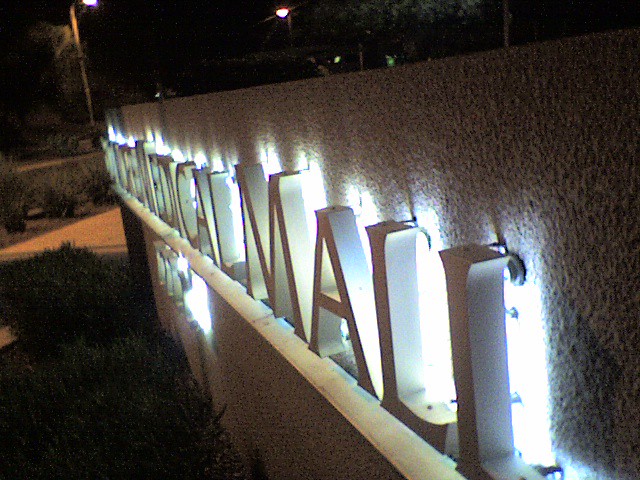This nighttime landscape photograph captures a lit sign on the facade of a stone wall in front of "The Medical Mall." The wall, a textured stone in a grey-white or apricot-light pink hue, serves as a backdrop to large, capitalized letters in a nude color. These letters are clearly visible due to the white LED backlighting shining on them. The wall stands about three feet above a well-maintained green patch of grass, with lush shrubbery and small bushes meticulously landscaped in front of it. Streetlights with warm white lights illuminate the scene, revealing a walkway and taller trees in the background. Although partially obscured, additional words on the wall suggest a larger message not fully captured in the image. The entire composition, from the lit sign to the surrounding greenery and urban elements, emphasizes the crisp, professional ambiance of the mall's exterior at night.